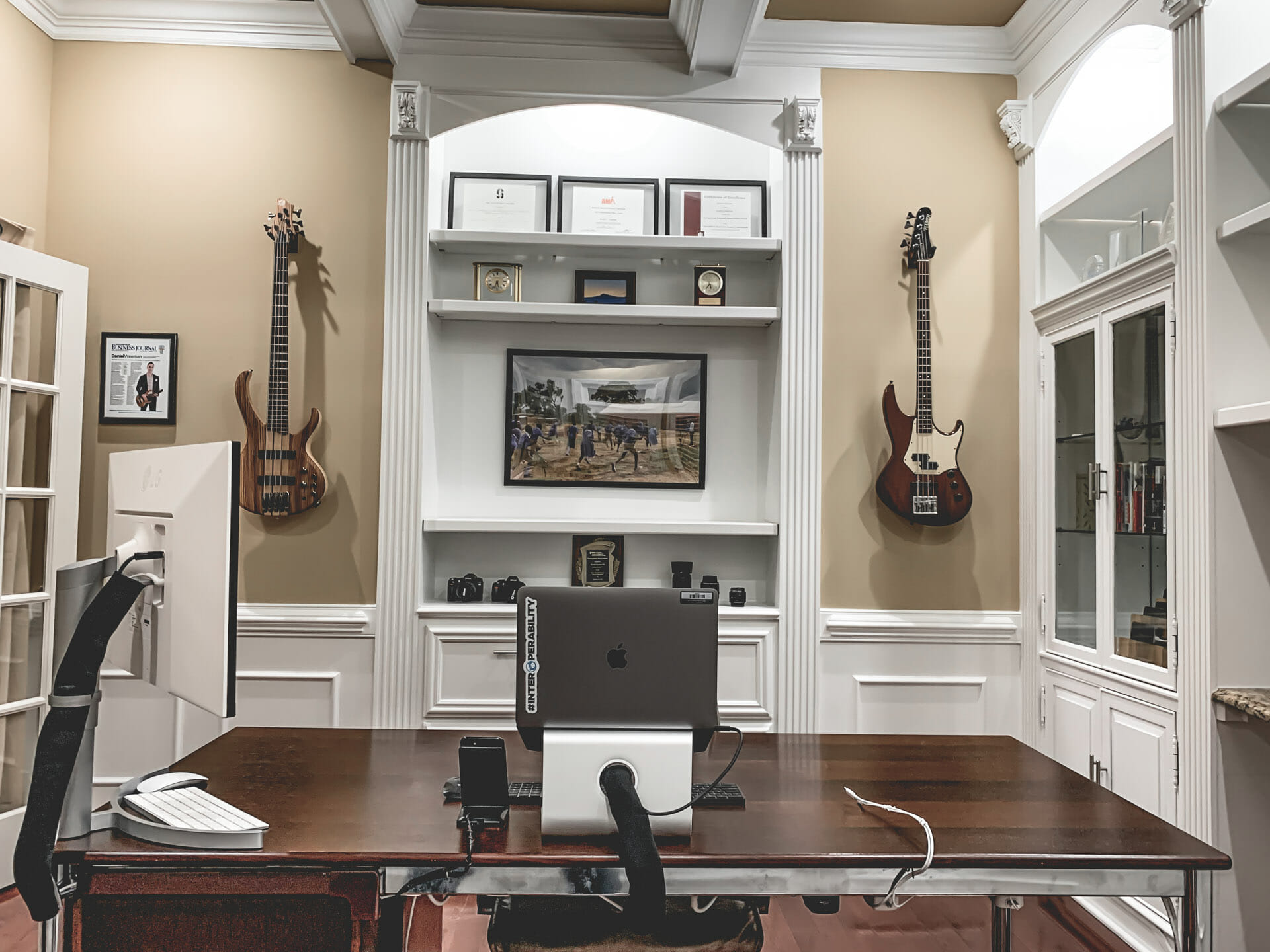The image depicts a well-organized home office or den with brown walls complemented by white trim on the cabinetry, floorboards, and door frames. On the left side, there's an open white wood and glass door. The central focus of the room is a white cutout wall adorned with multiple shelves displaying various photo frames, certificate plaques, awards, and cameras, indicating the occupant's interest in photography and achievements. Flanking this central section are two bass guitars: one with a brown wood body on the left and another with a tan and white body on the right.

In the far right-hand corner, a glass cabinet with white wood framing houses a collection of books, DVDs, or CDs. Central to the room is a wooden desk featuring a comprehensive setup: a white computer monitor and keyboard with a mouse on the left side and a black or gray laptop on a stand in the center, presumably a MacBook. A speaker and additional accessories are also present on the desk, making this a functional workspace.